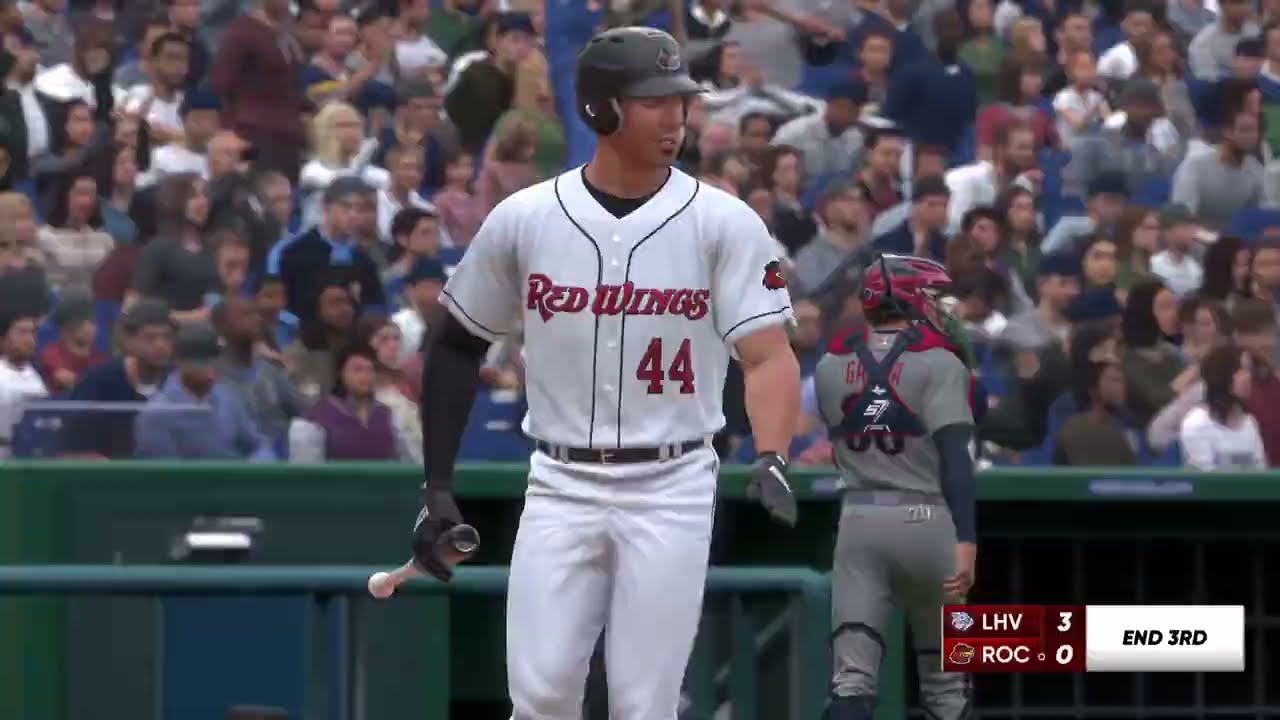The image portrays a professional baseball game, likely captured from a game broadcast or highlights reel. At the center of the image is a batter, wearing a white jersey emblazoned with "Red Wings" and the number 44, and matching white trousers. Positioned to the right and slightly behind the batter is the catcher, part of the opposing team, dressed in a grey uniform and red helmet. The stadium is filled with spectators, visible in the background, suggesting a lively game atmosphere. In the bottom right corner, a scoreboard indicates the score: LHV 3 - ROC 0, with a note that it is the end of the 3rd inning. The entire setting appears vibrant with colors like green, blue, white, red, black, and gray, and has a distinct appearance, reminiscent of a stylized video game graphic.